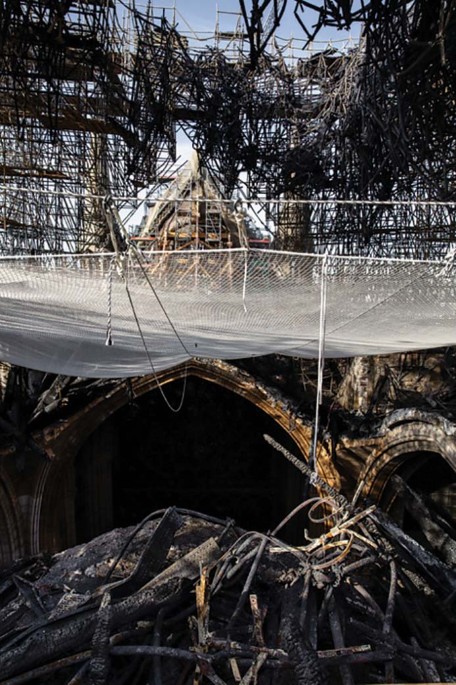The photograph depicts the ruins of a weathered structure, characterized by two prominent archways at the foreground. These archways, appearing rusted and aged, are topped with a ceiling composed of a chain-link fence or similar netting material. Piles of scrap metal, including bent rebar and rusted bars, clutter the ground in front of the arches, adding to the sense of decay. Above the arches, a chaotic tangle of collapsed rebar frames further accentuates the destruction. The upper portion of the image reveals a bit of blue sky, contrasting starkly with the derelict scene. The overall impression is of a once-sturdy structure now in disrepair, with numerous pieces of debris scattered all around. No text is present within the image to provide additional context.